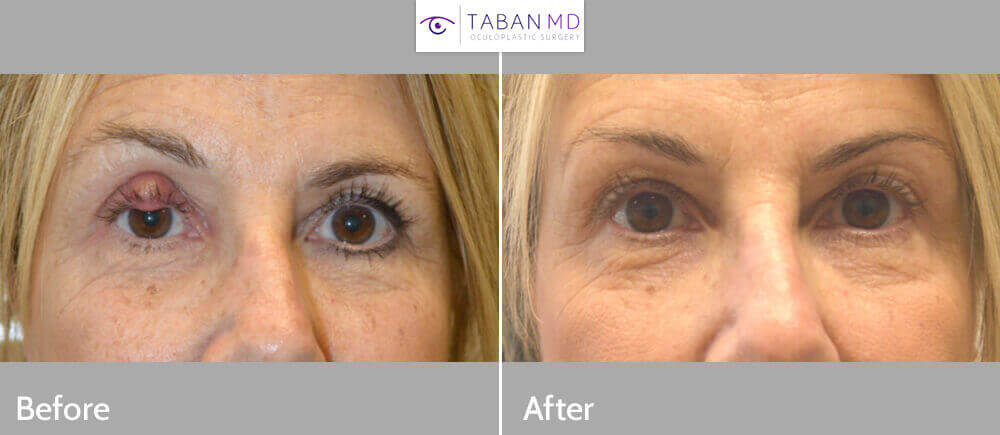The image features a before-and-after comparison of a middle-aged Caucasian woman with blonde hair, brown eyebrows, and brown eyes. The top of the image displays the text "Taban MD" in blue print, accompanied by a logo of an eye, and the phrase "Oculoplastic Surgery." The background at the top and bottom is a light baby blue. The left side of the image, labeled "before" in white font, shows the woman's face from the tip of her nose to her forehead, highlighting a noticeable protrusion, resembling a small pellet or massive stye, on her right eyelid partially covering her eye. The right side of the image, labeled "after" in white font near the center, shows the same woman after the removal of the eye protrusion, with both eyes appearing completely clear as she looks into the camera.